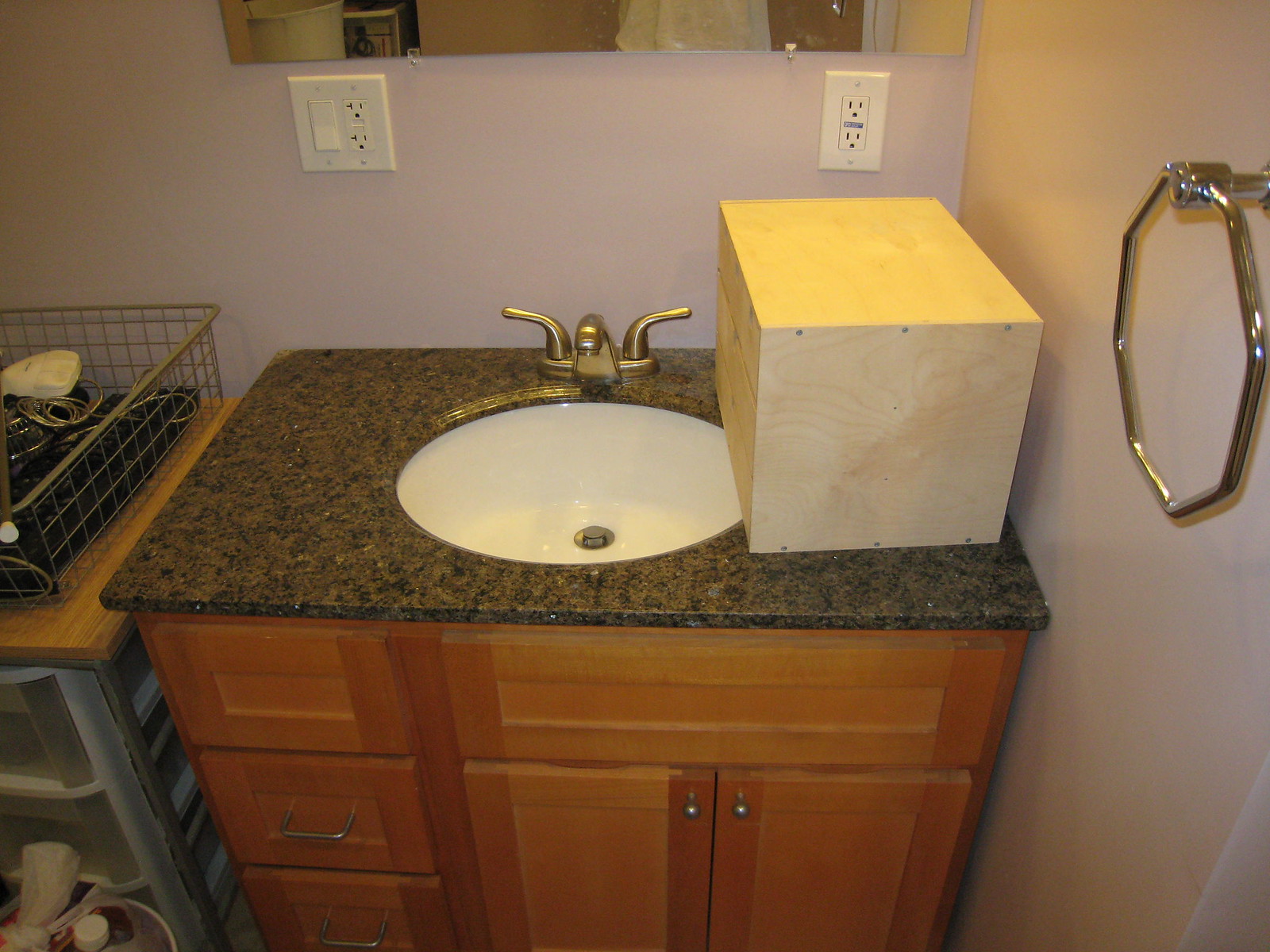A photograph of a basic bathroom showcases a simple yet functional vanity setup. The vanity features a sleek stone countertop, possibly marble, resting on a modest wooden base that includes several drawers. A wicker basket filled with assorted items is positioned beside the vanity, adding a touch of rustic charm to the otherwise straightforward décor. The sink, part of the vanity, is understated and juxtaposed with an oversized, plain pine wood box that sits precariously on the counter's edge, partially hanging over the sink area. 

In the image, a towel ring is visible but left empty, emphasizing the minimalistic aesthetic. Electrical fixtures include both a rocker switch and a standard outlet, contributing to the utilitarian feel of the space. The upper part of a mirror is cut off at the top edge of the photo, leaving its frame and size partially to the imagination.

The lighting in the room is provided by an overhead source from the top right, casting a yellow hue that somewhat distorts the true color of the walls. The walls themselves appear to be a muted gray or light lilac purple, though the yellowish tint softens and blends these tones into a warm blur in the photograph. Overall, this image captures a quaint, unembellished bathroom setting with a mix of muted colors and simple, functional furniture.